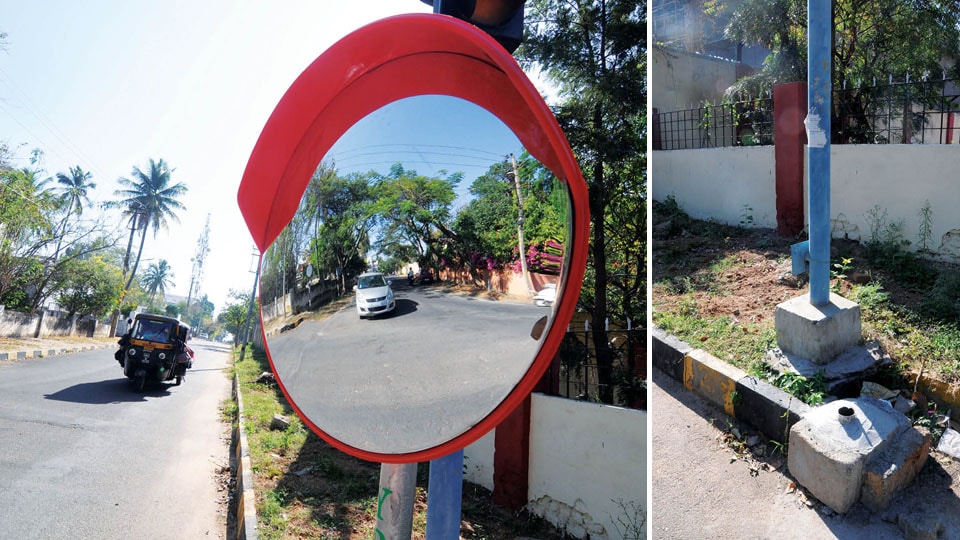The composite image is divided into two sections. The left section captures an urban street scene in what appears to be a Southeast Asian setting, with multiple palm trees visible in the distance. A large convex traffic mirror, mounted on a pole and edged with a prominent red border, is the focal point. Reflected in the mirror, one can see dense foliage and a white vehicle approaching. Additionally, there is a small local vehicle, such as a motorcycle or scooter, indicating the bustling street life typical of the region. The right section of the image shows a blue pole on a grassy verge adjacent to a street. This pole appears to be part of the traffic infrastructure, possibly associated with a traffic light. The base of a broken-off pole is also visible, surrounded by dirt and sparse vegetation, indicating it was once part of the same setup but is now missing. Near the pole, there is residue from an old poster and a cement fence nearby, likely delineating a residential area.